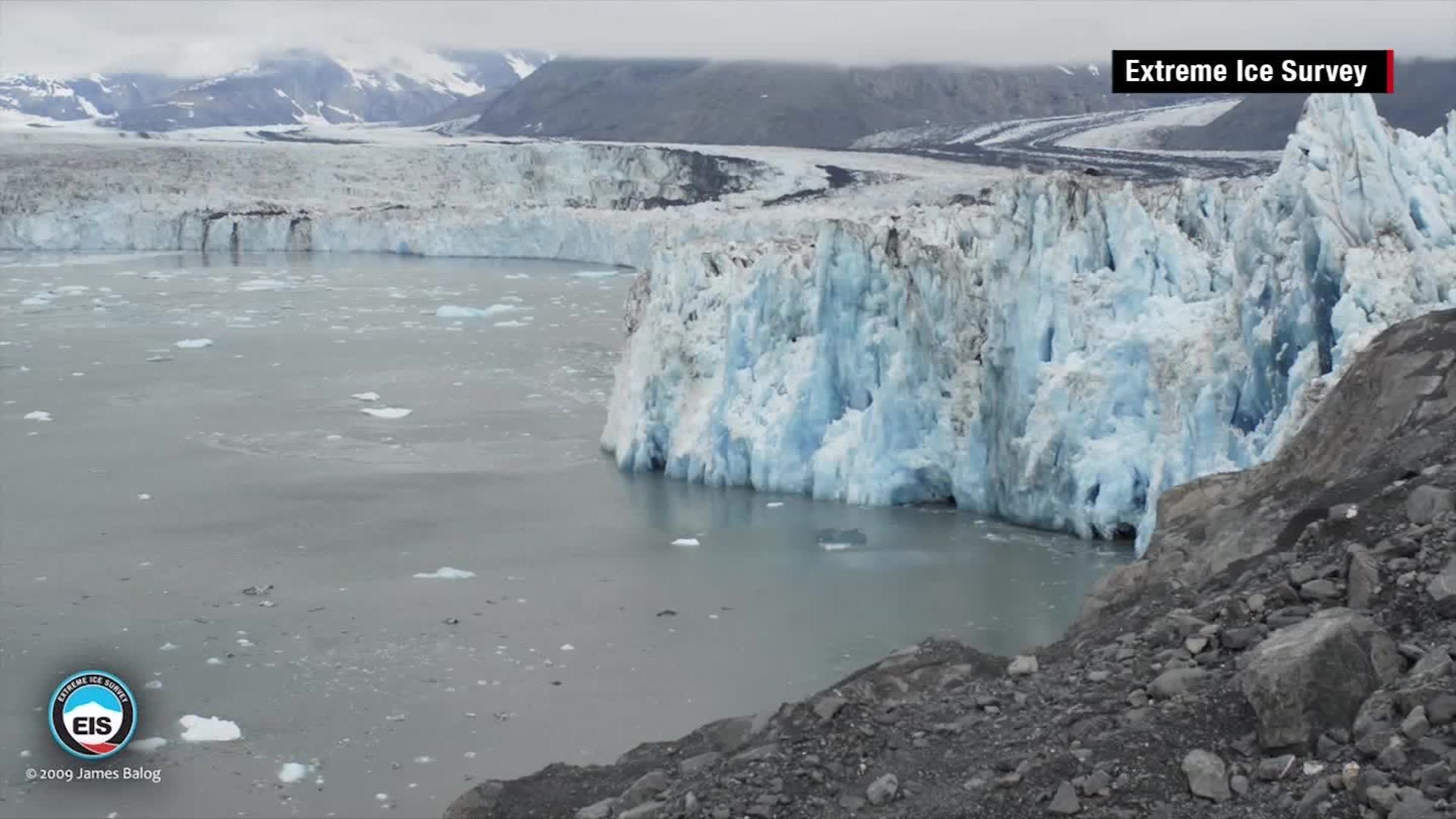This photograph, attributed to James Balogh in 2009 and marked with an "EIS" logo, captures a stunning panoramic view of a glacier, likely situated in Canada. The glacier, with its striking light blue ice, snakes its way through a valley, terminating in a body of still water—possibly a lake or ocean inlet. The icy formation, juxtaposed against a foreground of dark, almost volcanic-looking soil, creates a stark contrast in textures and colors. Small patches of floating ice dot the tranquil water's surface.

In the background, rugged mountains, some appearing flat-topped as if sliced by a knife, are partially snow-covered. These mountains serve as a dramatic backdrop to the glacier and contribute to the overall majestic landscape. The dirt in the foreground, predominantly dark and smeared with brown hues, extends to the right, while the left side of the image transitions into the serene water, lending a balanced composition to the scene.

Various other glaciers appear to cascade around a central mass of earth in the upper center portion of the photo, adding depth and complexity to the natural tableau. This eloquently layered landscape, devoid of any other identifying information, remains a testament to the raw and untouched beauty of glacial regions.